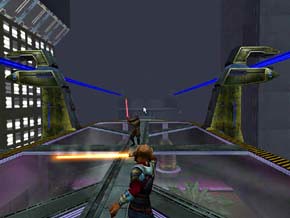The image is a widescreen freeze frame from a video game, depicting an intense lightsaber duel. Central in the scene, but slight off to the left, a figure with its back partially towards the viewer, stands ready. The left arm is foreshortened and visible, while the right hand firmly grasps a vividly yellow lightsaber held horizontally, extending to the left. 

Opposing this figure stands a dark-clad opponent, possibly Darth Vader, gripping a reddish-orangish lightsaber with both hands, poised for combat. The background exudes a high-tech aesthetic; the lower portion features a combination of steel and translucent materials with visible plants beneath. The left side of the scene is punctuated with illuminated panels, while the right side transitions into an industrial-looking structure that seemingly descends into an abyss. The overall atmosphere is charged with anticipation and high-stakes tension, capturing a climactic moment in the game.